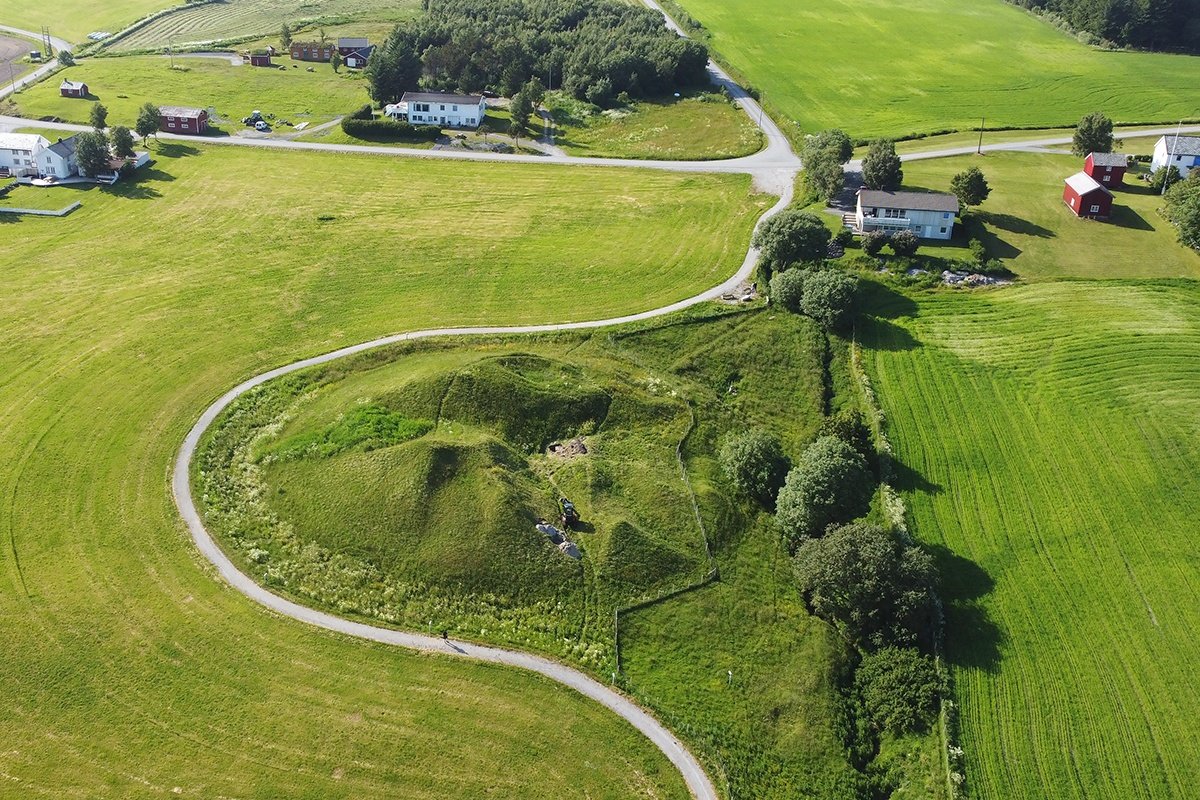This is an overhead aerial image of a quaint rural neighborhood or small town set amidst expansive green fields and rolling grassy hills. Predominantly, the landscape is divided into several plots of land, each adorned with lush greenery and interspersed with a variety of homes and agricultural structures. A large, winding gray road curves around the fields, originating from the upper left-hand corner and intersecting towards the upper portion of the photo before splitting and curling both upwards and downwards towards the bottom of the image.

The homes are a mix of sizes and styles, with some being large, multi-story edifices and others resembling smaller barns and sheds. Among them, several white houses with brown roofs stand out, with one notable two-story house featuring a gray outer structure beside red barns and a white and blue house with a gray roof on the right-hand side.

The center of the image showcases a particularly verdant area with darker green grass and a few scattered trees, adding to the picturesque charm. In the upper left-hand section, crops can be seen growing, reinforcing the agricultural essence of the area.

Overall, the image captures the essence of a serene countryside with a blend of residential homes, farm buildings, and extensive green areas, all connected by a winding road meandering through the vibrant landscape.